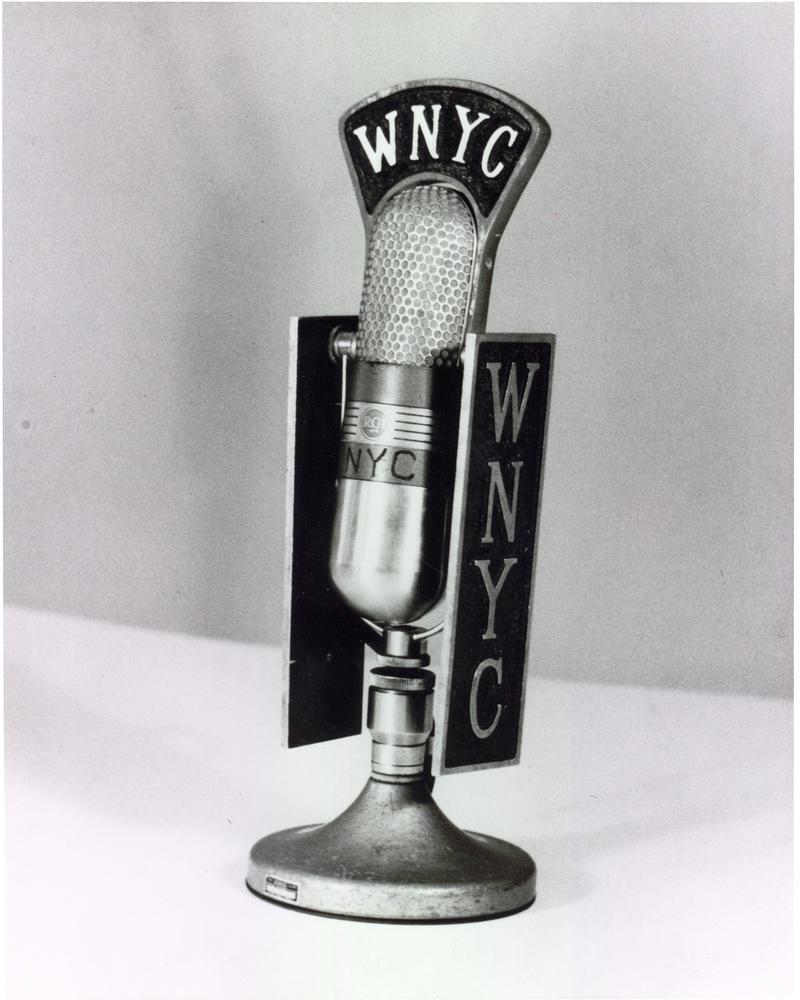This is a highly detailed black-and-white vertical photograph featuring a vintage microphone prominently placed at the center. The background comprises a white wall and a white surface, creating a stark contrast to the monochromatic and metallic tones of the microphone. The microphone, which appears to be made of heavy, likely stainless steel, is designed in a classic style reminiscent of the 1930s to 1960s era. The design includes a solid cylindrical body and a top section fitted with a mesh grill for sound capture, resembling a giant capsule or pill. Displayed on the microphone is the call sign "WNYC" in white font against a black background, visible at the top and on the sides. The microphone is mounted on a solid, round base, indicating it was possibly used on a desk, likely for radio broadcasting at WNYC. Though the microphone seems unplugged, hinting it is currently on display, its robust build suggests it was made for durability and long-term use.